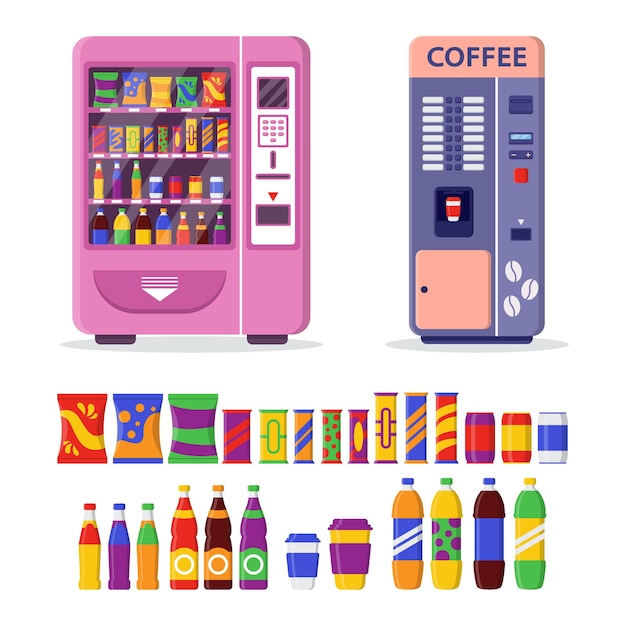The image features two computer-generated cartoon vending machines on a white background. The primary machine is a vibrant purplish-pink, offering a selection of chips, candies, and various kinds of drinks displayed over its four shelves. The top two shelves showcase assorted snacks, while the bottom shelves contain sodas in an array of bottles and cans, some featuring bubbly polka dot designs to indicate carbonation. A white panel with a code punch system and a downward-pointing arrow guides users to retrieve their selections. Adjacent to this is a smaller, tan and gray coffee vending machine with blue text reading "COFFEE" at the top and adorned with white coffee bean illustrations. The machine has a prominent orange door with a black knob where users collect their customized coffee cups. Below the machines, the snacks, drinks, and two cups of coffee—available from the coffee dispenser—are enlarged and meticulously arranged for clear visibility.